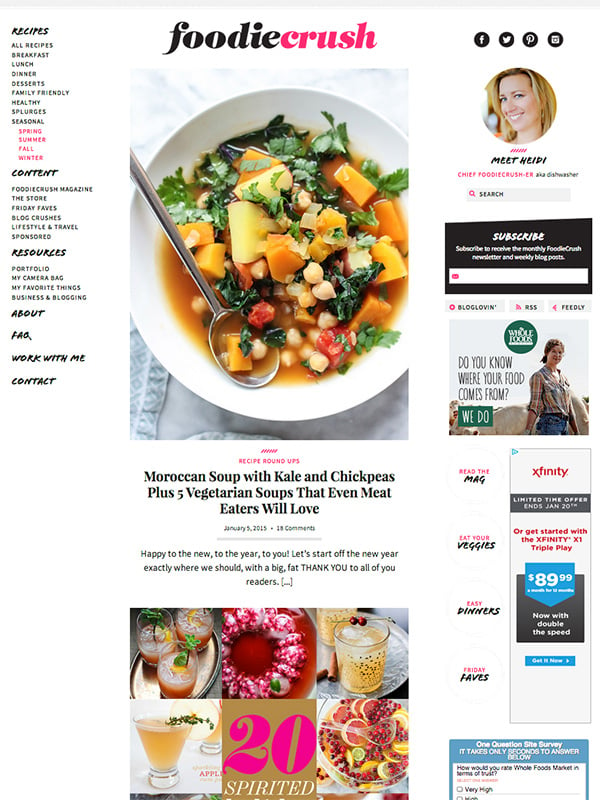The rectangular image, oriented vertically, appears to be a screenshot from a website or app divided into three columns. 

The left-hand column features a comprehensive menu bar. Top to bottom, this menu is segmented into different categories: "Recipes" with subcategories such as All Recipes, Breakfast, Lunch, Dinner, Desserts, Family Friendly, Healthy, Splurges, and Seasonal. Under "Seasonal," written in red, the options are Spring, Summer, Fall, and Winter. Following, in italicized bold, "Content" includes Foodie Crush Magazine, The Store, Friday Faves, Blog Crushes, Lifestyle & Travel, and Sponsored. Lastly, "Resources" provides links to Portfolio, My Camera Bag, My Favorite Thing, Success in Business and Blogging, About, FAQ, Work With Me, and Contact.

The middle column prominently displays the website's title, "Foodie Crush," accompanied by an enticing image of a bowl filled with a hearty vegetable soup—possibly Moroccan with kale and chickpeas. The title beneath the image reads, "Moroccan Soup with Kale and Chickpeas Plus Five Vegetarian Soups That Even Meat Eaters Will Love." Below this are a series of other images, arranged collage-style, hinting at additional content.

In the right-hand column, a photograph likely depicting the site’s author is visible, along with various advertisements—the most recognizable being for Xfinity.